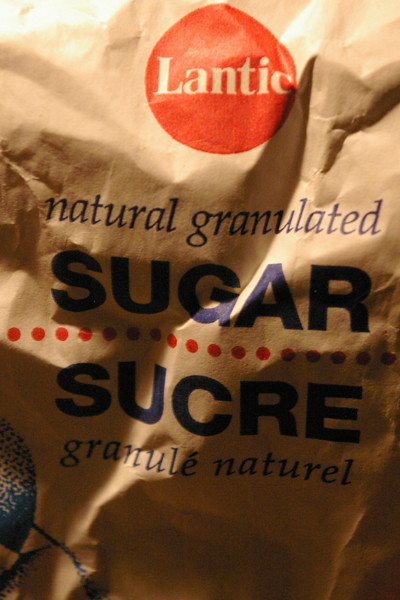This image showcases a partially crumpled brown paper bag, its surface marred by numerous wrinkles. Prominently displayed in the top-middle section of the bag is a solid red circle with the brand name "LANTIC" inscribed in white letters. Below this red circle, the words "naturally granulated" stand out in dark blue font, followed by a larger "SUGAR" inscription in bold blue capital letters. Centrally placed red polka dots divide the English text from its French counterpart—"sucre granule naturel"—also written in blue text. The bag bears signs of lighting variance, highlighting certain sections more brightly than others, while some parts remain in shadow. An additional detail includes an image that is partially cut off at the bottom left, and a round blue and white mark can be seen on the left-hand side of the bag.